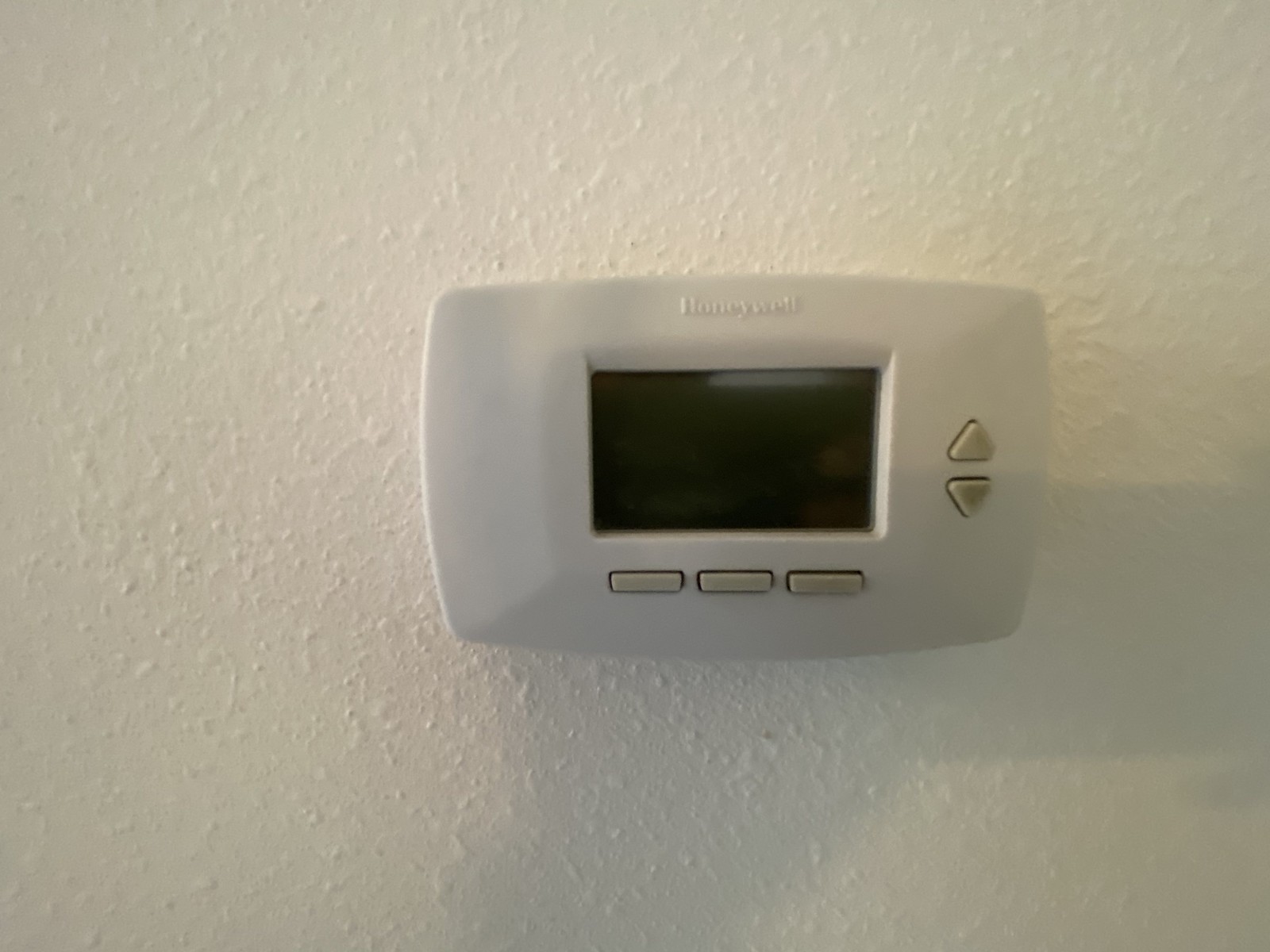In this photograph, we see a textured white wall with a slightly uneven surface featuring subtle bumps. Mounted on this wall is a Honeywell thermostat. The device, made of plastic, has a rectangular shape with a black, unlit screen positioned in the center. Above the screen, the brand name "Honeywell" is raised in a distinct font. Below the screen, there are three elongated, gray rectangular buttons. To the right side of the screen, there are two additional gray buttons: an up arrow and a down arrow, presumably for adjusting the temperature. The thermostat appears somewhat dirty, suggesting it could be quite old.